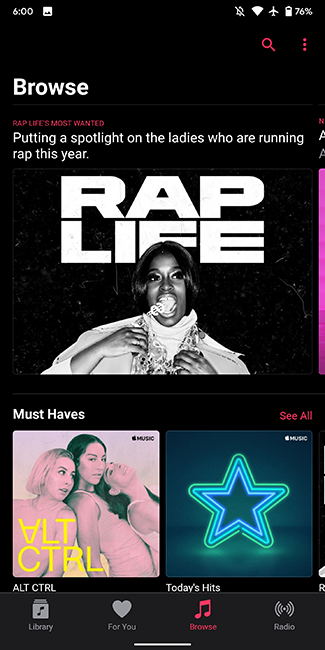This is a detailed screenshot captured on an Android device precisely at 6 o'clock. The device shows full Wi-Fi connectivity, Airplane Mode activated, the ringer on silent mode, and a battery level at 76%. In the top right corner, there is a red search arrow and three vertical dots indicating more options.

The interface displays features such as an option to browse or explore more songs. The bottom of the screen includes a red "Browse" label accompanied by a radio icon. Adjacent to this, there are additional options for discovering more songs. On the bottom left, there is a small icon for the Music Library. Centrally positioned at the bottom, a heart icon signifies the area where users can save their favorite music.

In the middle of the screen, there appears to be an image possibly of Alicia Banks, a singer, with "Rap Life" written prominently behind her. She is depicted with her mouth open, emitting dollar signs. Beneath this, three women are shown leaning against one another with "Control" written alongside, indicating a music album cover. Various other icons and details are scattered across the interface, enhancing its functionality and aesthetic appeal.